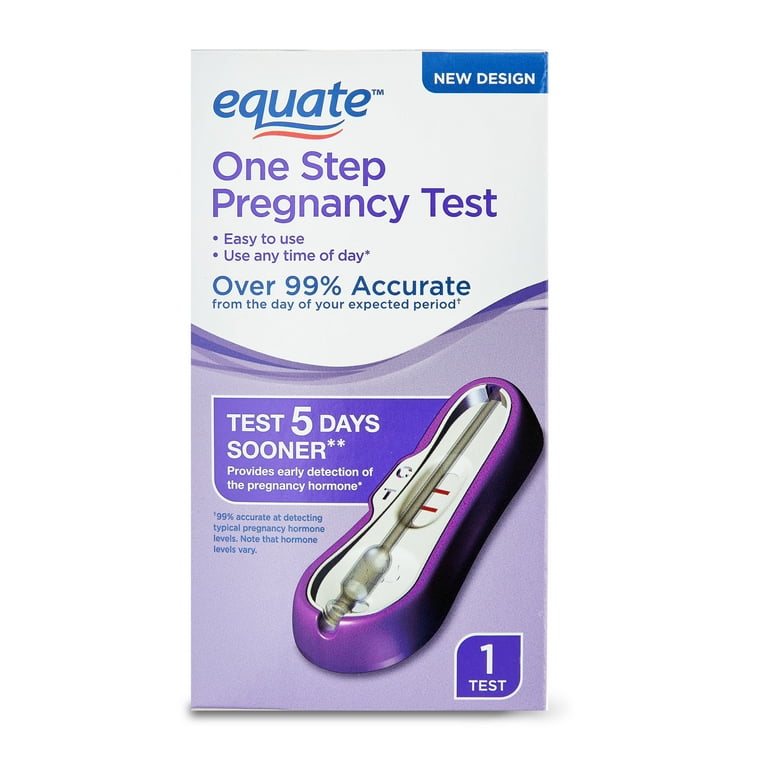This image displays a rectangular box of Equate’s one-step pregnancy test, featuring a new design. The majority of the box is white with purple sections at the top and bottom, and it also incorporates some blue accents. The brand name “Equate” is written prominently in navy lettering. A blue box in the upper right corner of the packaging states "New Design." The text on the box highlights the key features: it is easy to use at any time of the day, over 99% accurate from the day of your expected period, and capable of testing five days sooner by providing early detection of the pregnancy hormone. Additionally, the text emphasizes that the test is 99% accurate at detecting typical pregnancy hormone levels, but notes that hormone levels can vary.

The packaging also includes an image of the pregnancy test, which is purple and white, with a depiction of two red lines that indicate the test results. The test device features the letters "C" and "T" on its side and contains some blue writing. The box includes one test and is likely photographed in a store setting given the focus on the product box.